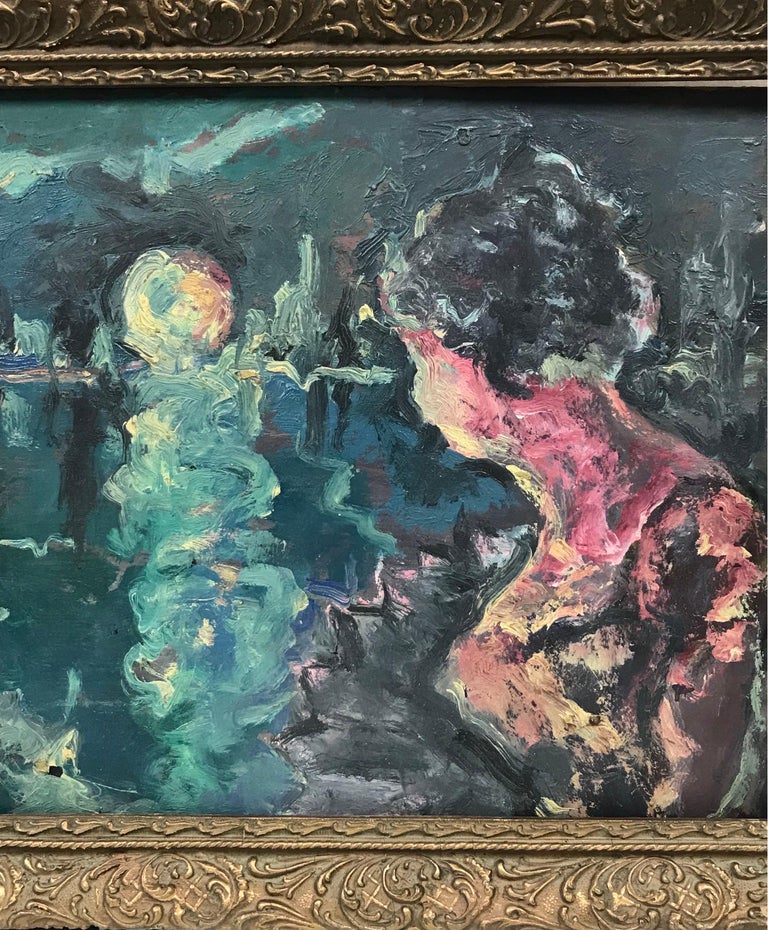This photograph showcases a framed painting with a distinctly abstract aesthetic. The painting is set within a classic, articulated gold frame, where only the top and bottom edges are visible, creating a bordered effect. The main subject of the piece is a woman viewed in profile, gazing backwards towards what might be the reflection of the moon over a body of water, framed by a cityscape or landscape that remains ambiguous due to its abstraction.

The woman's neck and the side of her face are highlighted with deep pinks and reds, while her hair appears dark. She seems to be wearing a dress that incorporates shades of red, gray, and yellow, blending into the color palette of her flesh tones. The background behind her consists of murky and heavy brushstrokes with a dominant greenish hue, alongside splashes of gold and yellow-green, creating an impressionistic feel similar to German Expressionist works. The texture of the paint is thick, adding to the painting's rough and expressive character. Overall, the prominent colors in this evocative piece are gold, blue, red, and green, creating a striking juxtaposition of hues and forms.